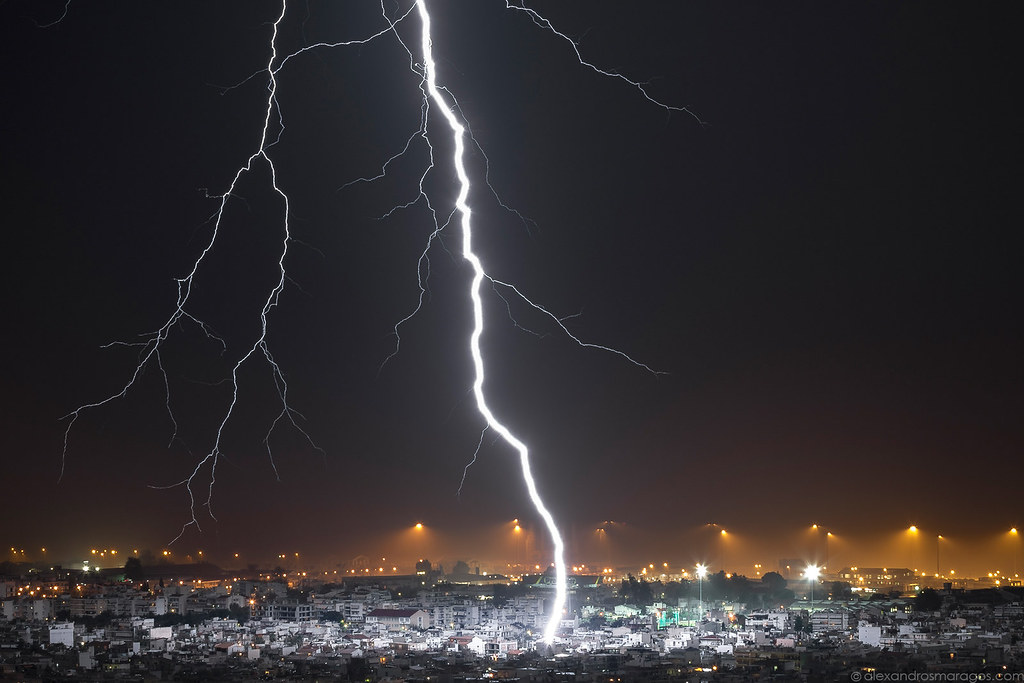This color nighttime photograph captures a dramatic moment where a vivid lightning bolt strikes a sprawling cityscape from a distance. The dark black sky provides a stark contrast to the brilliant white lightning bolt, which dominates the left half of the image, branching out like tree roots as it extends downward. The main bolt, jagged and intense, touches down in the city, highlighting apartment buildings, skyscrapers, and other structures with its powerful glow. The lightning's luminosity overshadows details of the buildings, casting them in a bright but somewhat indistinct white light. Scattered forked lightning bolts accompany the main strike, adding to the scene's complexity. Below the dark sky, the city is illuminated by a combination of amber-hued streetlights and the pervasive city lights, indicating the robust nightlife of a city comparable in size to New York. Toweringly tall street lamps, possibly lining a freeway, contribute to the yellowish light that intermixes with the ambient glow from homes, businesses, and other urban fixtures.